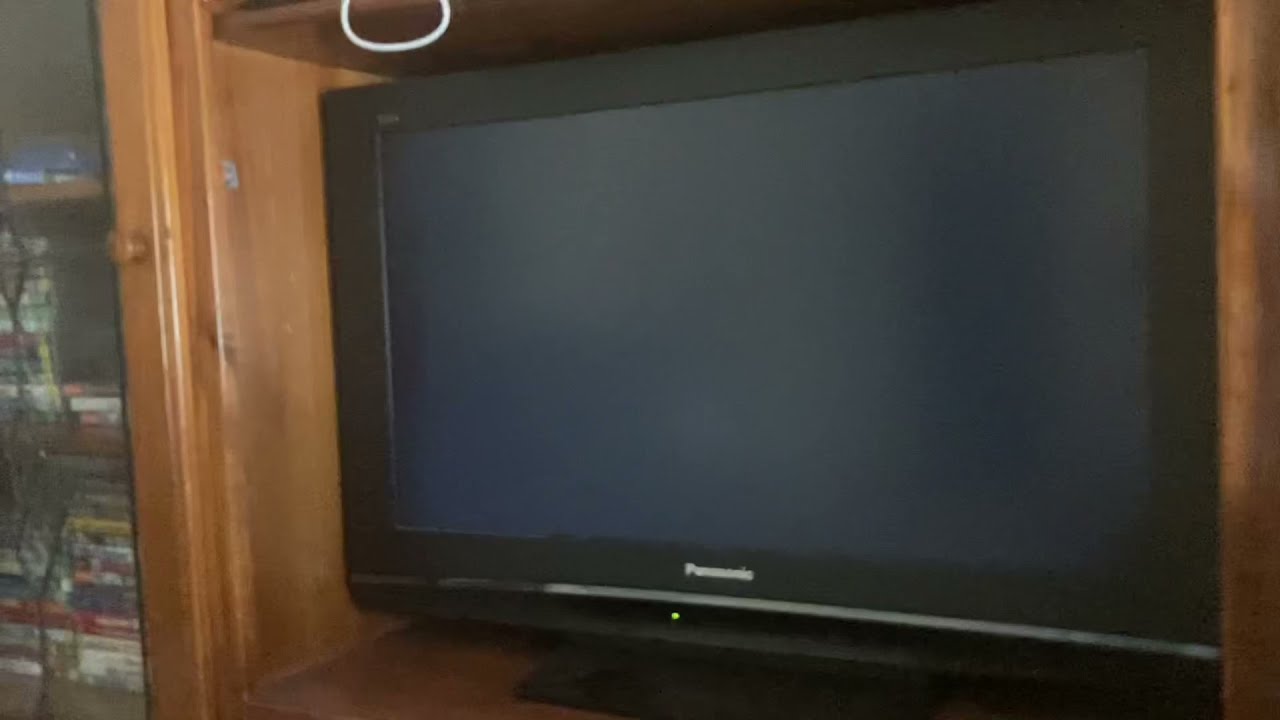The image depicts a vintage Panasonic monitor placed at the center within a brown wooden shelving unit. The screen of the monitor is turned off. To the left of the monitor, there is a CD/DVD rack filled with discs. Notable colors in the image include brown, black, gray, red, light green, purple, and white. At the top of the shelf, there's a small loop, and a green button can be seen beneath a section where it seems to say "panoramic." The setting appears to be indoors, suggesting an older photo, likely from the early 2000s, perhaps taken in a hotel room.